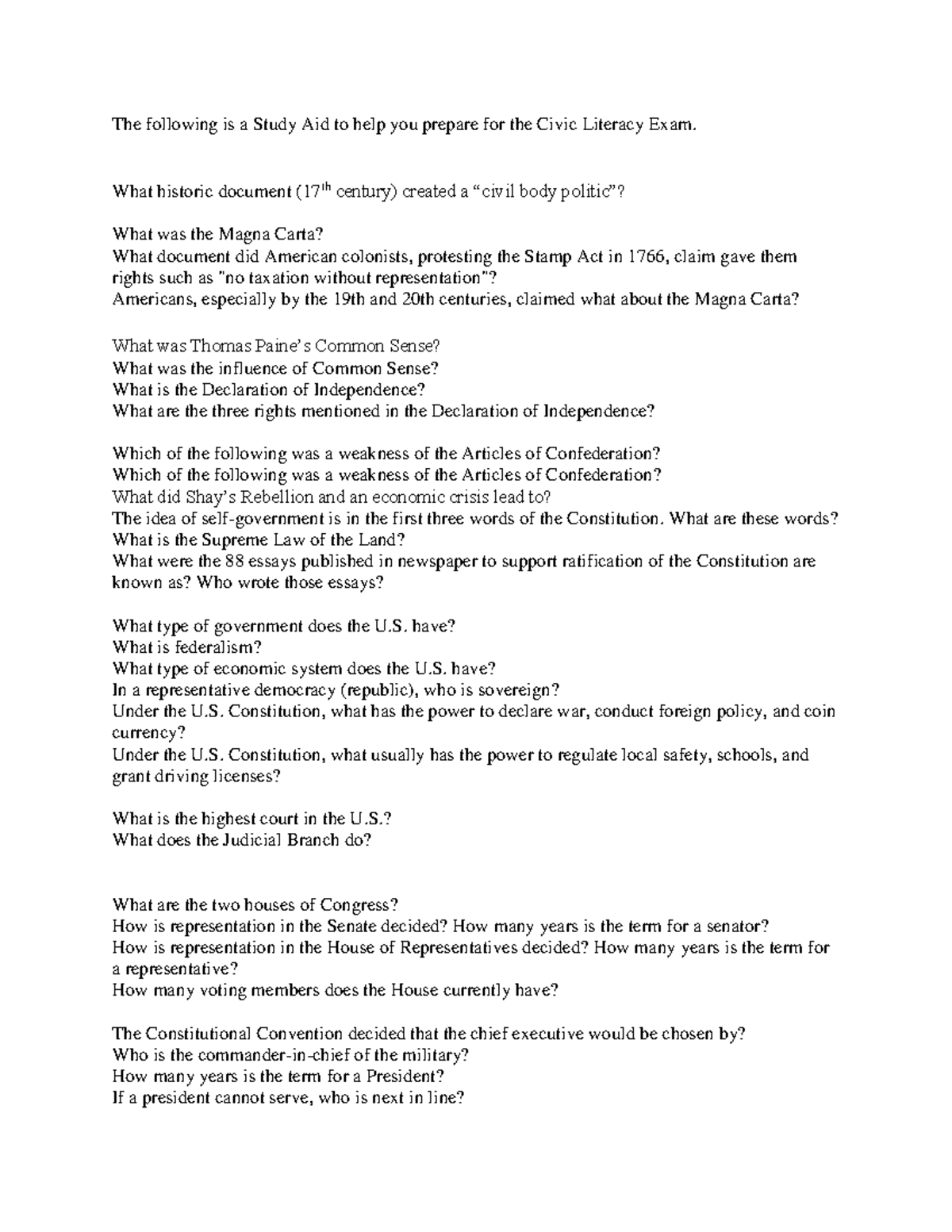The image consists of several lines of small black text organized as a study aid for the Civic Literacy Exam. At the top, a capitalized heading reads: "STUDY AID TO HELP YOU PREPARE FOR THE CIVIC LITERACY EXAM." Below the heading, the text is structured as a series of historical and governmental questions aimed to aid in exam preparation.

The first question asks, "What historic document (17th century) created a 'civil body politic'?" followed by the inquiry, "What was the Magna Carta?" in question format. It continues with another historical question: "What document did American colonists protesting the Stamp Act of 1766 claim gave them rights such as 'no taxation without representation'?" 

Moving deeper into American history, the text includes a question reflecting on the 19th and 20th centuries: "Americans, especially by the 19th and 20th centuries, claimed what about the Magna Carta?"

Following these, the text presents a series of questions about the United States Congress. The second-to-last paragraph reads:
- "What are the two houses of Congress?"
- "How is representation in the Senate decided?"
- "How many years is the term for a senator?"
- "How is representation in the House of Representatives decided?"
- "How many years are the terms for a representative?"
- "How many voting members does the House currently have?"

The final paragraph consists of four questions, with the last question asking: "If a president cannot serve, who is next in line?"